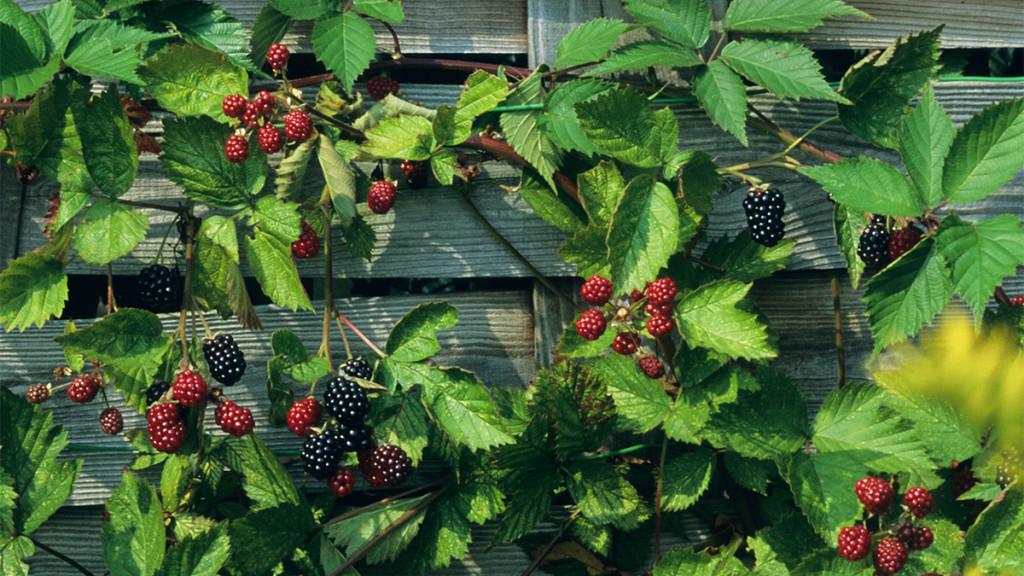The photograph captures a lush wall of leaves, predominantly green with some turning yellow at the bottom, draped over a fairly weathered gray lattice or wooden fence. The greenery is dense, overshadowing the lattice, but glimpses of the aged wood are still visible. Among the dark and light green foliage are numerous clusters of raspberries and blackberries at various stages of ripening. Some berries are a deep purple, indicating they are nearly ripe, while others are an immature red. The vines and branches wrap around the fence, creating a tapestry of leaves and fruit. Each berry cluster typically contains about six to seven berries, adding to the abundant feel of the plant. Shadows behind the leaves suggest the photo was taken midday, further highlighting the textures and colors of the scene.